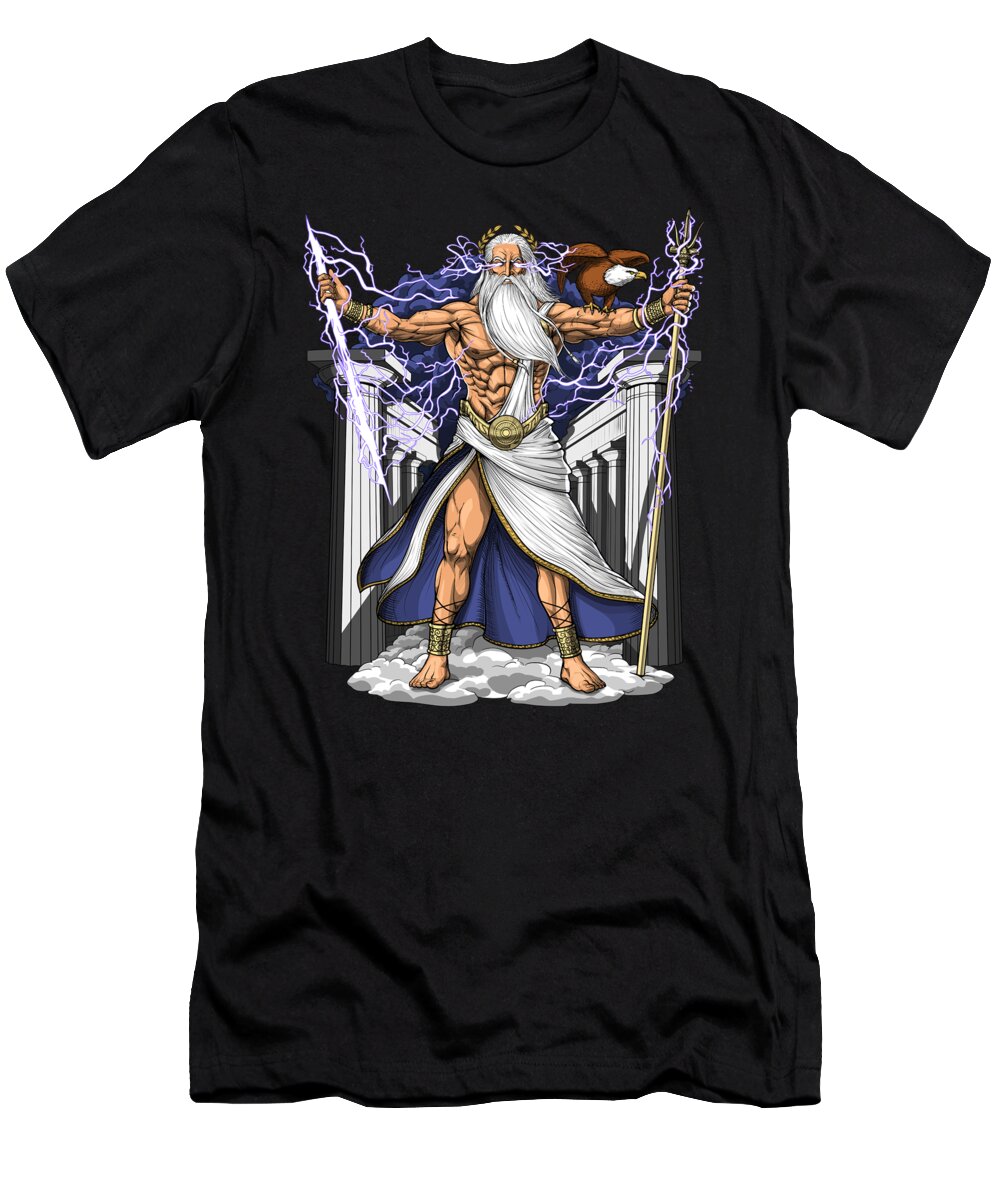This is a detailed color photograph of a short-sleeved black cotton t-shirt, displayed on a white background, perfect for online shopping. The t-shirt features a large screen-pressed graphic that spans from the shoulder area down to about the belly button. The central design showcases a tall and imposing Zeus, the Greek god, who is depicted with long flowing white hair and a lengthy beard. He is bare-chested, revealing his highly muscular torso and arms, and is wearing a white toga with a rich blue interior draped around his lower body.

Zeus is depicted barefoot, with cuffs around each ankle. In his right hand, he wields a thunderbolt radiating with lightning, and in his left hand, he holds a scepter that emits electrical lines connecting to the thunderbolt. Zeus is crowned with a laurel wreath, emphasizing his godly status. Adding to the powerful visual, a majestic eagle is perched on his left bicep, facing right and gazing at the electrified scepter. Behind Zeus, the backdrop includes white columns receding into the background and more lightning illuminating the sky, creating a dramatic and electrifying scene.